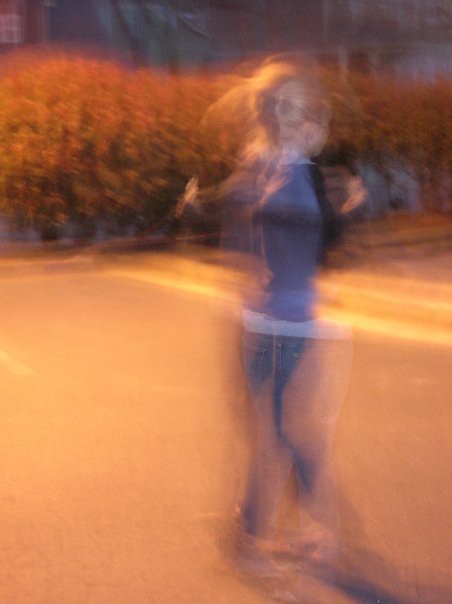In the foreground of this blurry image, a woman stands in a parking lot, surrounded by faint glares that obscure finer details. She appears to be wearing a blue top with a white collar, and her blonde hair is neatly tied up in a bun. She also seems to be dressed in blue jeans. Behind her, white parking spot lines are visible, adding context to the setting. Further in the background, a horizontal row of bushes spans the scene, beyond which an apartment building is discernible. The top left corner of the image includes a glimpse of a small brick structure, juxtaposing the greenery. The overall atmosphere hints at a residential area, captured in haste or possibly at a distance.